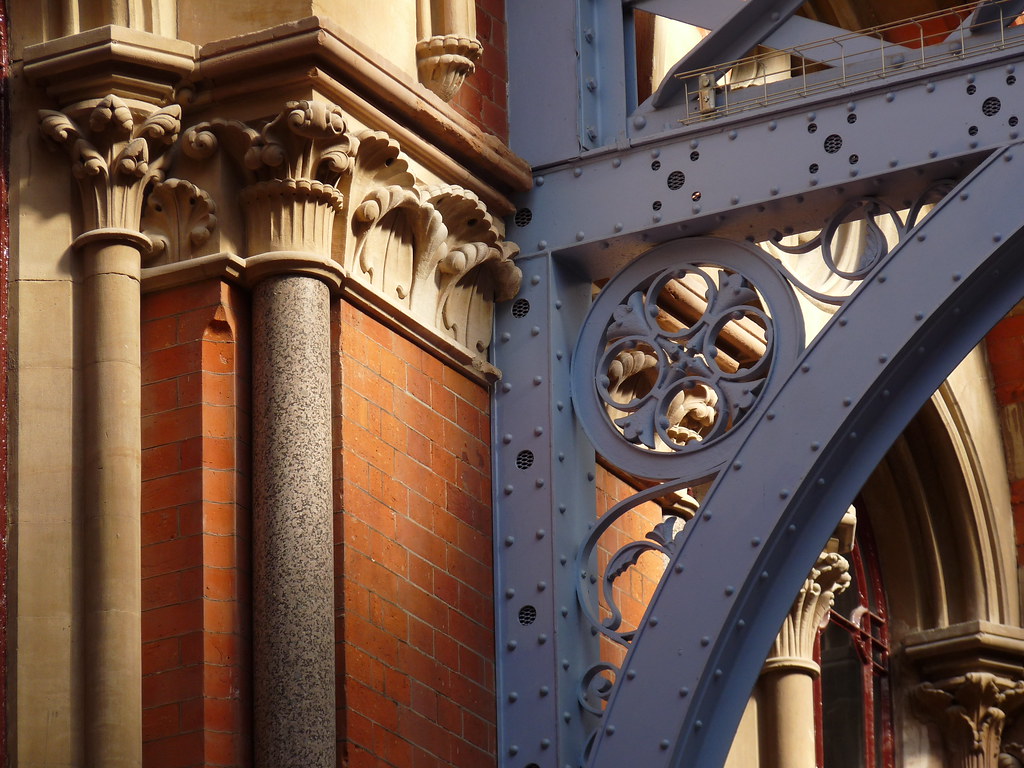The photograph showcases a detailed side view of a historic building characterized by a blend of old and new elements. The main structure is constructed from brown bricks, featuring intricate neoclassical columns and trim possibly made of cement, giving the facade a dignified, antiquated appearance. On the left side, one column stands out with a gray stucco finish and beige or off-white trim, adorned with various designs leading up to arches at the top. The right side of the image prominently displays a modern metallic framework, painted gray, possibly steel or iron, which intersects with the brickwork. This metallic structure includes numerous screws and studs, and mimics the gothic design of the original brickwork in an attempt to harmonize the old and new architectural styles. A notable element is a large door with a rounded arch visible at the lower right. Above the metallic framework, additional scaffolding can be seen, contributing to the complex layers of design present in the facade.